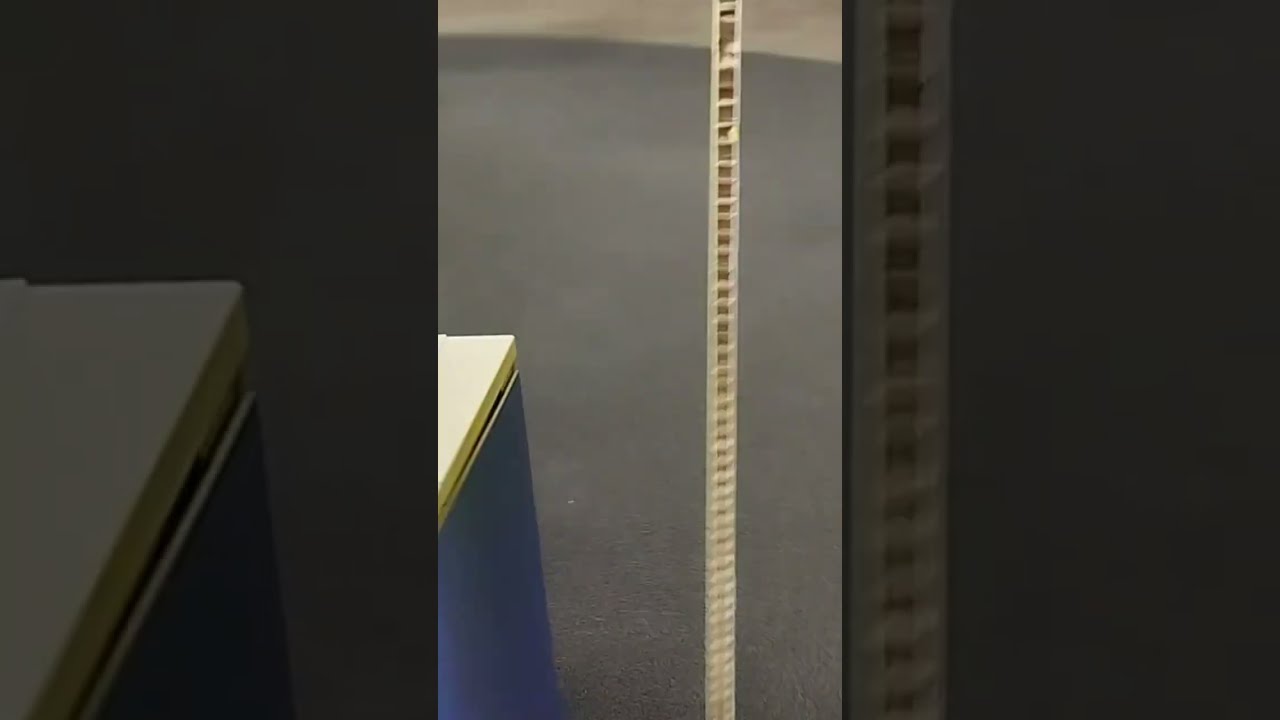This vertical photo, possibly a video still, depicts a detailed close-up of the corner of a blue cabinet or desk with a light-colored top, potentially made of wood or formica, set against a gray carpet background. Dominating the central portion of the image is a tall, slender structure resembling a small, handmade ladder—possibly crafted from balsa wood or a tape-like material. This stack has numerous horizontal rungs, estimated to be around 40, creating a repetitive pattern from the bottom to the top of the photo. The photo is oriented in portrait mode, encapsulated within a landscape frame necessary to fit the broader space. The left and right sides of this frame are filled with opaque black overlays that blur and obscure some details, adding a darker gray tint and magnified effect to those sections without detracting from the main vertical elements of the image.